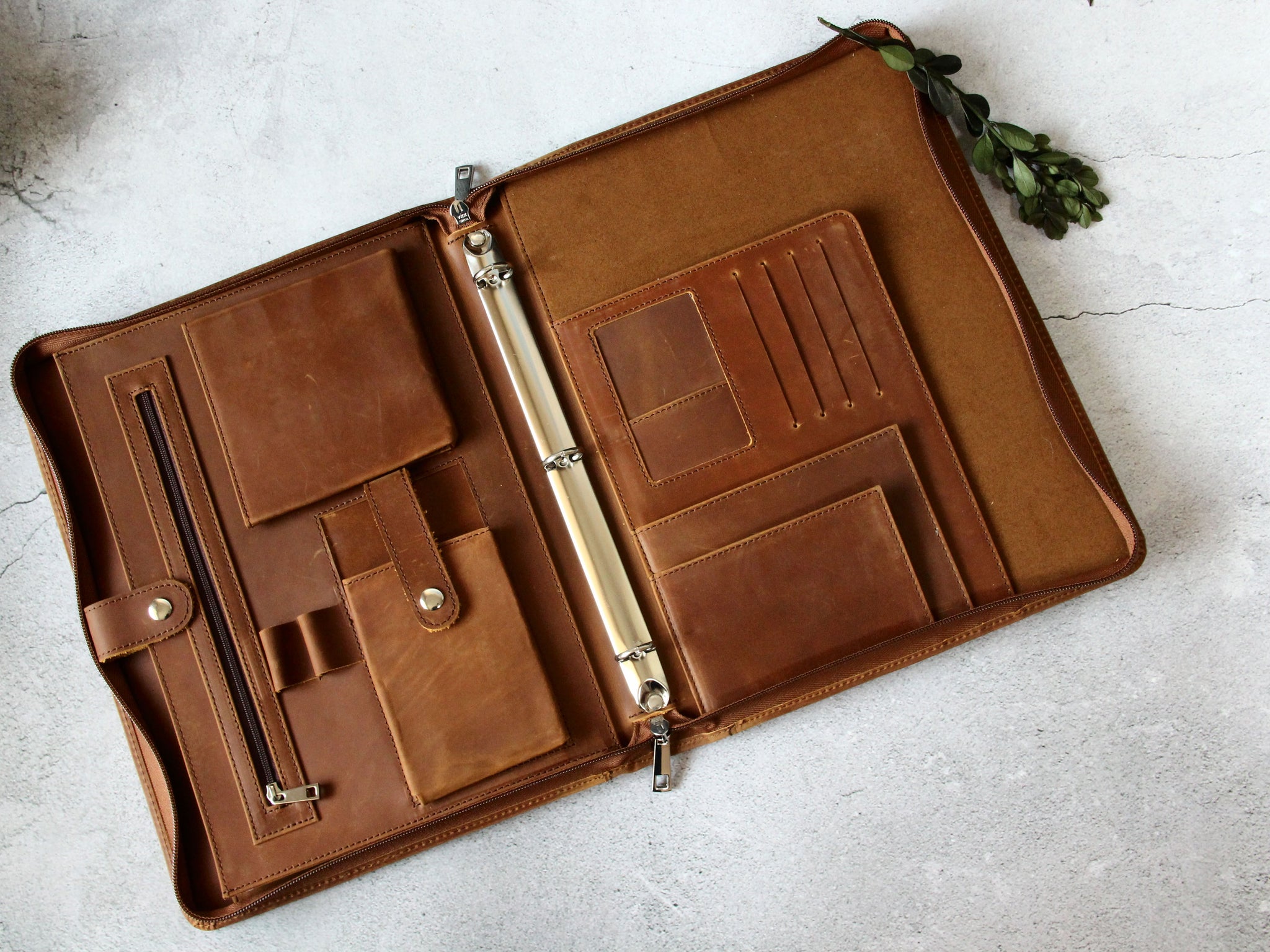This image showcases a detailed brown leather carrying case taking up the majority of the frame, approximately 70%. The leather case exhibits different shades of brown and is adorned with multiple compartments secured by a variety of closures including snaps, buckles, and zippers. On the left side, there is a zipper and buckle that, when opened, reveal additional spaces designed to carry various items. Centrally located, a white zipper with a silver handle provides access to more storage, possibly for papers or a tablet, and adjacent compartments offer yet more organizational features, likely suitable for phones, documents, and even a three-ring binder.

In the upper right corner of the photo, a green plant with several leaves adds a touch of nature against a background of a white wall marked with visible cracks on both the left and right sides of the image. The setting appears to be indoors, potentially captured for a catalog or a website aiming to showcase the multifunctional aspects of the carrying case, which could also serve as a journal, notebook holder, or wallet.